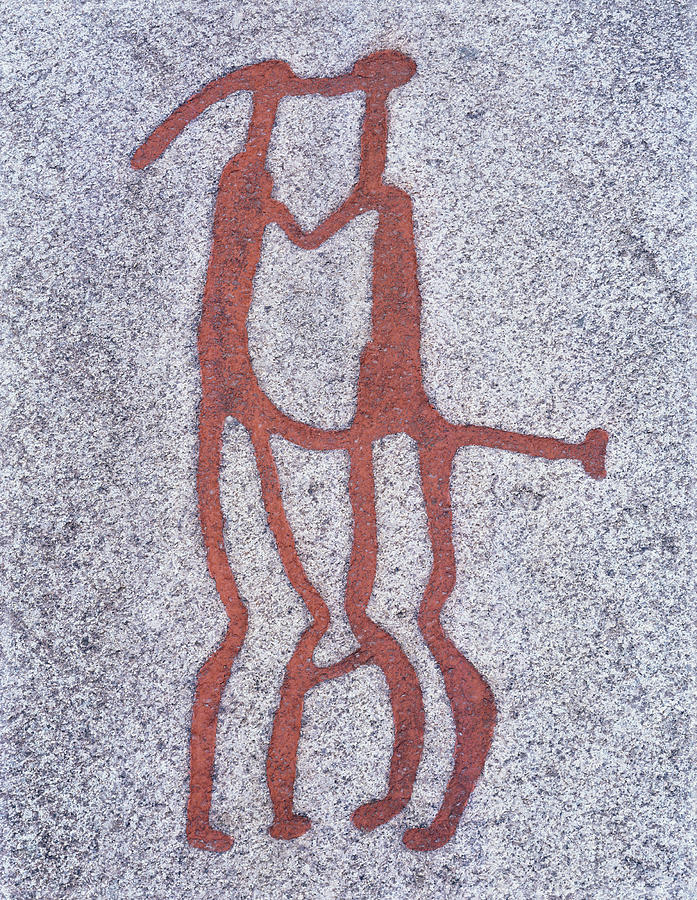The image depicts an ancient prehistoric cave painting or engraving on a gray, pitted stone tile, marked with flecks of black. The artwork, characterized by thin, wispy lines of dark copper or red paint, portrays two elongated, nondescript figures standing upright. These figures appear to be intertwined and embracing, joined at the shoulders, hips, and knees. One figure has a tail, while the other seems to wear an elongated headdress. Its abstract nature leaves room for individual interpretation, suggesting it could either represent an expression of human or animal forms or a symbolic piece of art. The stone’s intricate and possibly historic design gives it a dual possibility of being a valuable museum artifact or a creative representation.